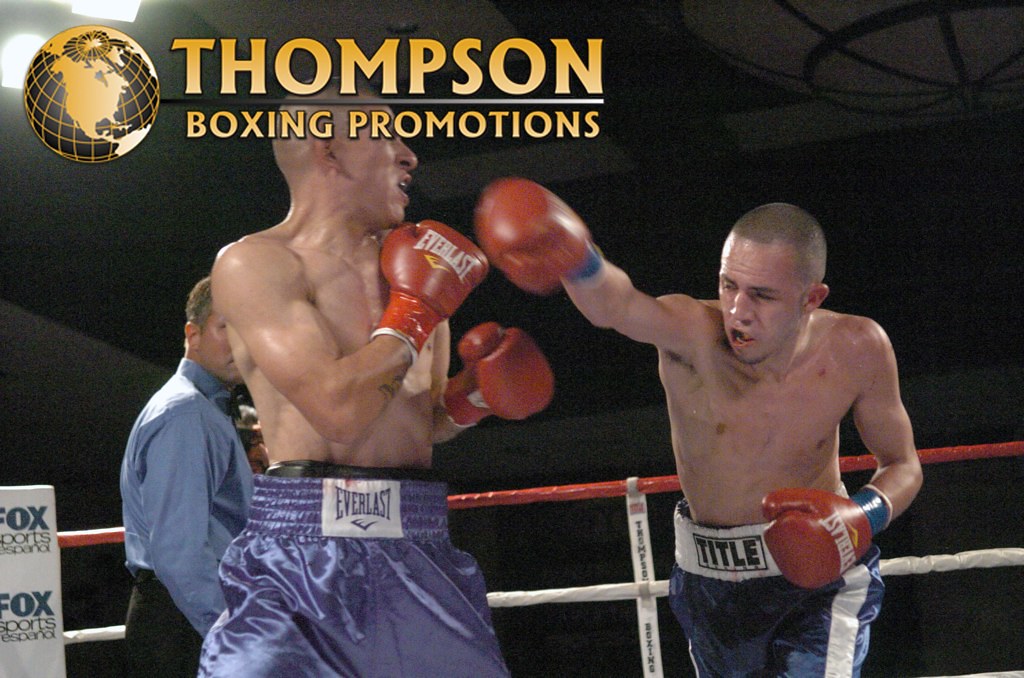In this detailed photograph taken inside a boxing ring, the black background prominently features the logo "Thompson Boxing Promotions" in gold text, accompanied by a gold-globed graphic of the world in the upper left-hand corner. A white box labeled "Fox Sports Español" is visible in the lower left-hand corner. 

Central to the image are two muscular, shirtless boxers with closely shaved heads, sporting identical red Everlast boxing gloves. The boxer on the left, wearing distinctive gray Everlast shorts, has both elbows bent defensively at about 60 degrees. In contrast, the boxer on the right, clad in dark blue Title shorts with a white stripe, is mid-action, delivering a punch with his right arm fully extended towards his opponent. 

Behind the boxers, the attentive referee, dressed in a long-sleeve blue shirt, black slacks, and a bow tie, watches the match closely. The ropes of the ring, marked by red and white stripes, frame the dynamic scene, completing this intense snapshot of athleticism and competition.